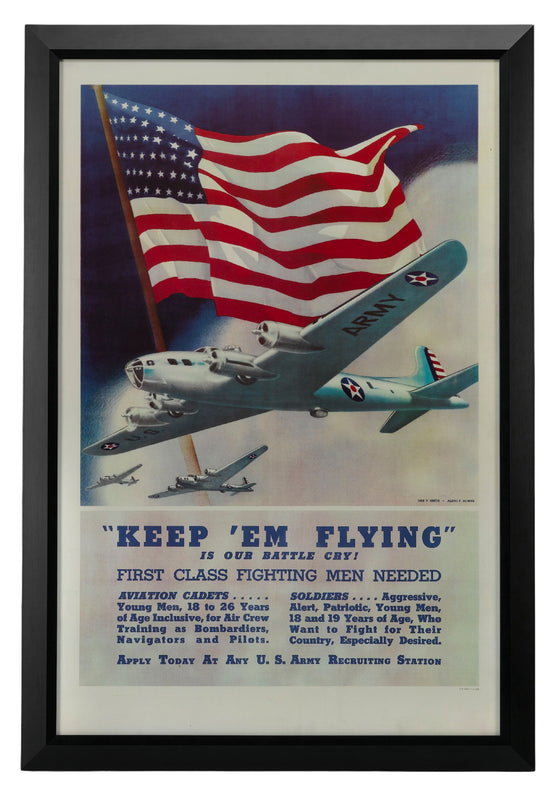This framed, color poster is a historical U.S. Army propaganda piece, likely from World War II. The artwork, which may be a gouache illustration, features three army planes labeled "Army" soaring across a deep blue sky partially filled with a large white cloud. An American flag waves in the background, reinforcing the patriotic theme. The poster prominently displays the bold, capitalized text: "Keep Them Flying is Our Battle Cry. First-Class Fighting Men Needed." It calls for young men, ages 18 to 26, to join as aviation cadets, including roles as bombardiers, navigators, and pilots, with a particular emphasis on alert, aggressive, and patriotic young men aged 18 and 19. The text finale urges these potential recruits to "Apply today at any U.S. Army Recruiting Station." The entire illustration and message are enclosed within a sleek black frame against a white background.